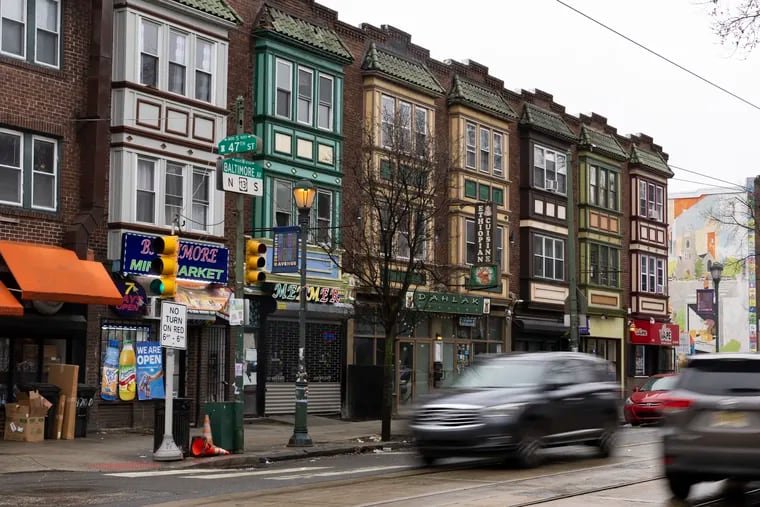In an overcast urban scene, a full-color photograph captures a small town street intersection, identified by green street signs marking 47th Street and Baltimore Avenue. The rectangular image, devoid of specific borders, features blurred cars, including an SUV, moving along a blacktop road that occupies the lower right section. On the left side, a series of three-story brick row houses with wood facades line the street. Each building's upper two floors house apartments, marked by rectangular windows, some with green tiled overhangs. The ground floors are street shops, including one with a prominent purple and pink storefront sign for a market named "Baltimore Mini Market" located in the second row house. Adding to the detailed urban landscape, there are green streetlights, a gray sidewalk, and bare tree branches with a power line visible in the top right corner. An additional touch of local color is provided by a mural on a building on the far right of the photo, promoting a vibrant yet homely street atmosphere.